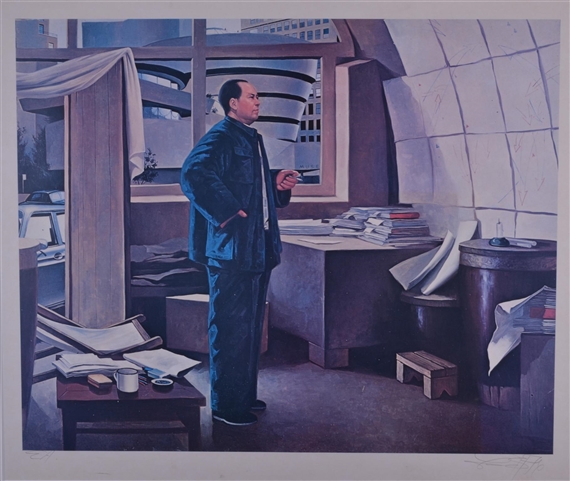This detailed painting portrays a man standing in what appears to be a modernist apartment or possibly a studio. He has dark, receding hair and a light complexion, and he wears a blue jacket along with matching blue pants over a white shirt. His left hand is balled into a fist at his stomach height, while his right hand is casually tucked into his jacket pocket. The man faces right with a solemn expression, contemplating something off-frame.

The room is gray and features a desk cluttered with books and papers to the man's right. A stool and a barrel also occupy the space, with a low table to his left holding a white mug and other small objects, possibly a deck of cards. The wall behind him is covered with a grid-like pattern filled with papers, creating an impression of meticulous disorder.

Behind the man, large windows span the back wall, revealing a cityscape dominated by a distinctive building with a spiral design, identified as the Guggenheim Museum. This inclusion, along with the man's dress and surroundings, subtly suggests he might be an artist or someone in a creative profession, standing thoughtfully in his somewhat disorganized yet inspiring creative space.